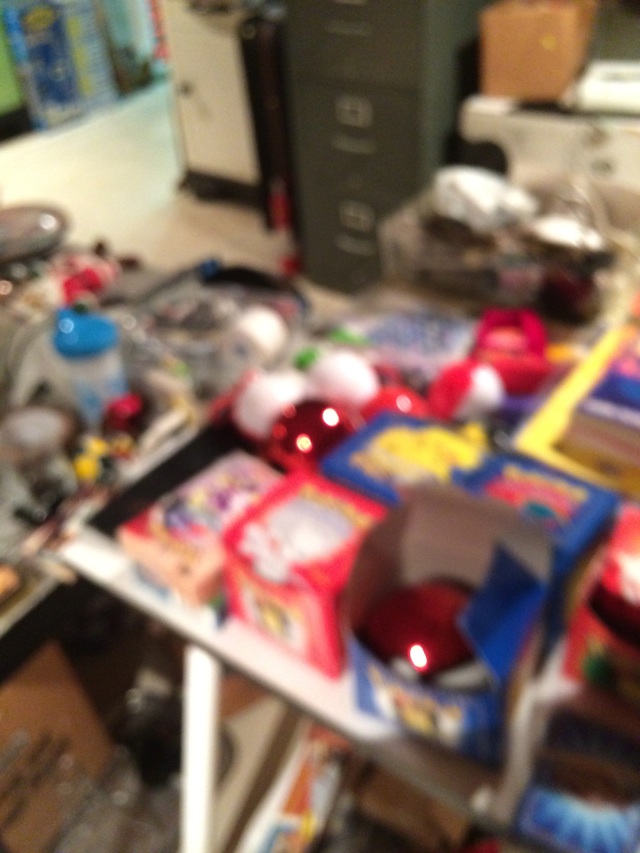The photograph, despite being very blurry, depicts a cluttered and jumbled scene that resembles a yard sale or a setup for a swap meet. Dominating the foreground is a large table covered with a disarray of items, including a prominent Pokeball from Pokémon, various children's toys, old tech gadgets like phones and answering machines, and Christmas ornaments, notably in red and white colors. Additionally, there are multiple plastic containers and knickknacks, adding to the impression of an eclectic assortment. In the background, a gray metal filing cabinet with silver handles and a white safe can be seen, hinting at an office-like environment. The floor is white tile, further suggesting an indoor setting. To the far left, there's a yellow table which holds books and magazines. Other miscellaneous items such as cuddly toys and a roll of toilet paper are also scattered around, enhancing the overall sense of organized chaos.